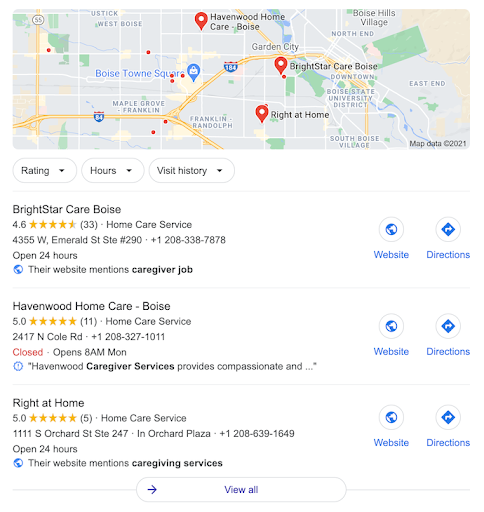This is a webpage designed for finding addresses or businesses, prominently featuring a map at the top. The map includes several highways and markers for specific locations. Below the map, there are several tabs labeled "Rating," "Hours," and "Visit History," all in black text.

The webpage highlights three specific home care services:

1. **Bright Star Care Boise**:
   - The name is in black text followed by its star rating.
   - A brief description of the service.
   - The address, phone number, and "Open 24 hours" are listed.
   - On the right, blue icons for the website link and directions are displayed.

2. **Havenwood Home Care Boise**:
   - The name is followed by the rating and a description as a home care service.
   - The address and operational hours are specified.

3. **Right at Home**:
   - The name is followed by the rating and described as a home care service.

The webpage has a white background with primarily black text, while the star ratings are gold and certain elements, including some text and icons, are blue. At the very bottom, there is a "View All" option with an arrow pointing right. The map at the top of the page marks the locations of the three services mentioned—Bright Star Care Boise, Havenwood Home Care Boise, and Right at Home—with red circle markers featuring a white center, indicating their exact locations.